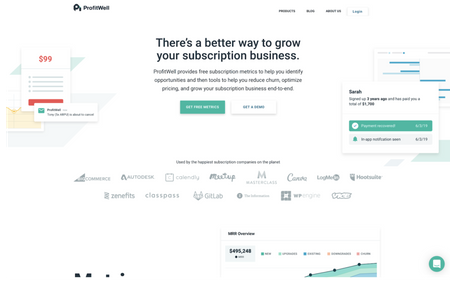The image features a central slogan that reads: "There's a better way to grow your subscription business." It highlights that ProfitWell provides free subscription metrics to help identify opportunities, reduce churn, optimize pricing, and grow subscription businesses end-to-end.

On the left side, there's a figure of $99 accompanied by descriptive text and a red checkmark. Below this, additional text proclaims that these services are "used by the happiest subscription businesses on the planet."

Logos of several well-known companies are displayed, including Commerce, Autodesk, Calendly, Meta, Masterclass, Logly, Zenefits, ClassPass, GitLab, and WP Engine. A partial logo and text hint at another company related to "Skill Overview," alongside a figure of $495,248. A chart is also present, providing a visual representation of metrics.

In the top right corner, there's a user profile summarizing that Sarah signed up three years ago and has generated a total revenue, though the exact figure is not specified.